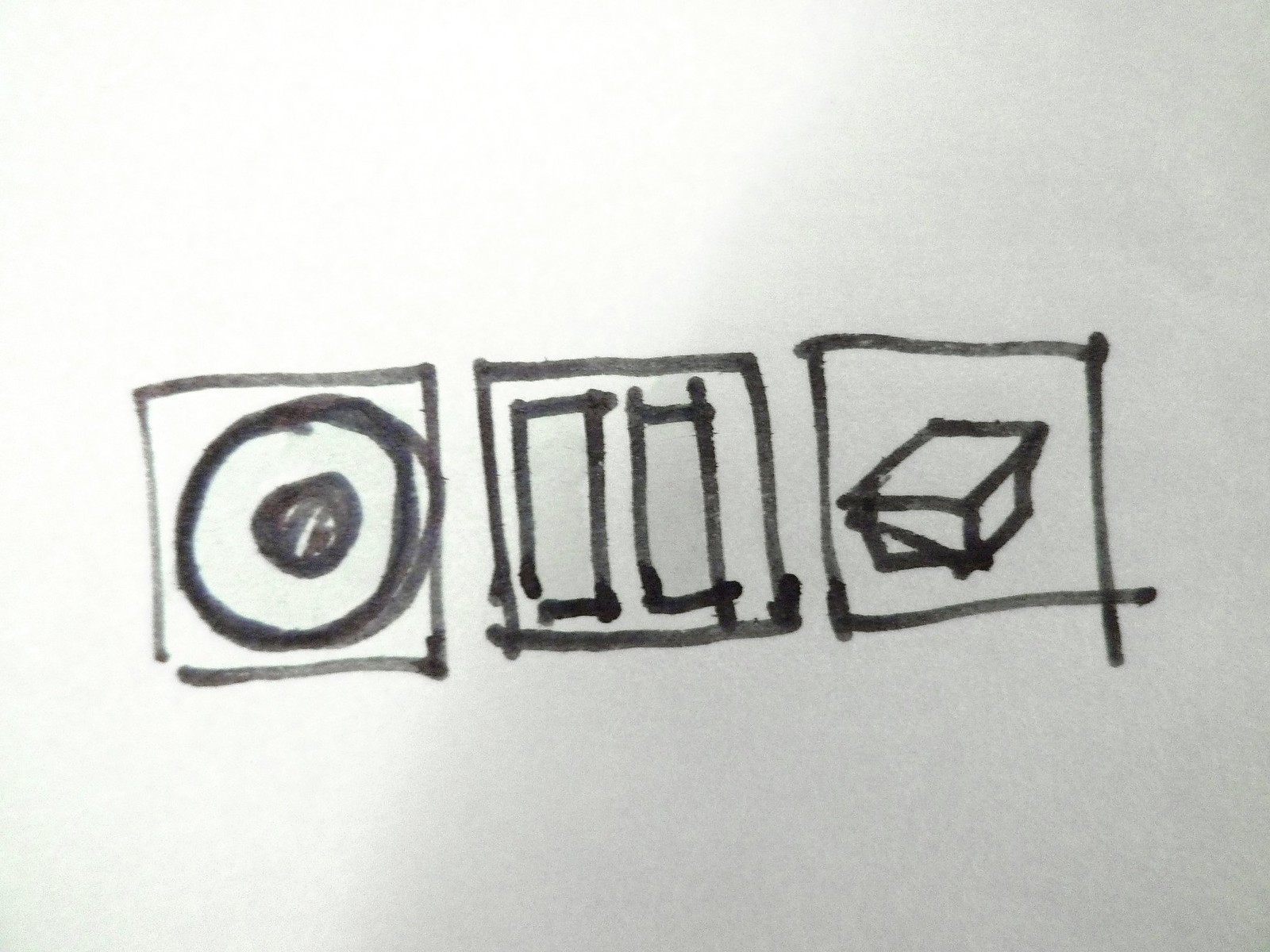The image displays three hand-drawn squares arranged horizontally in a row across the center of a piece of white paper. These drawings, rendered in black ink presumably from a Sharpie marker, have bled through to the side of the paper being observed. 

In the first square, a hollow circle is drawn, with another solidly colored circle of approximately two centimeters in diameter nestled inside it. 

The middle square contains two empty rectangles, also drawn in black ink, which are positioned side by side within the square's boundaries.

The third and final square features a three-dimensional rectangular prism. This prism has a diagonal line that appears to represent a handle, suggesting a way to lift or interact with the shape. Notably, the bottom line of the prism extends beyond the left boundary of the square, and the right side of the prism extends downward past the square's lower boundary, resulting in an overlapping effect.